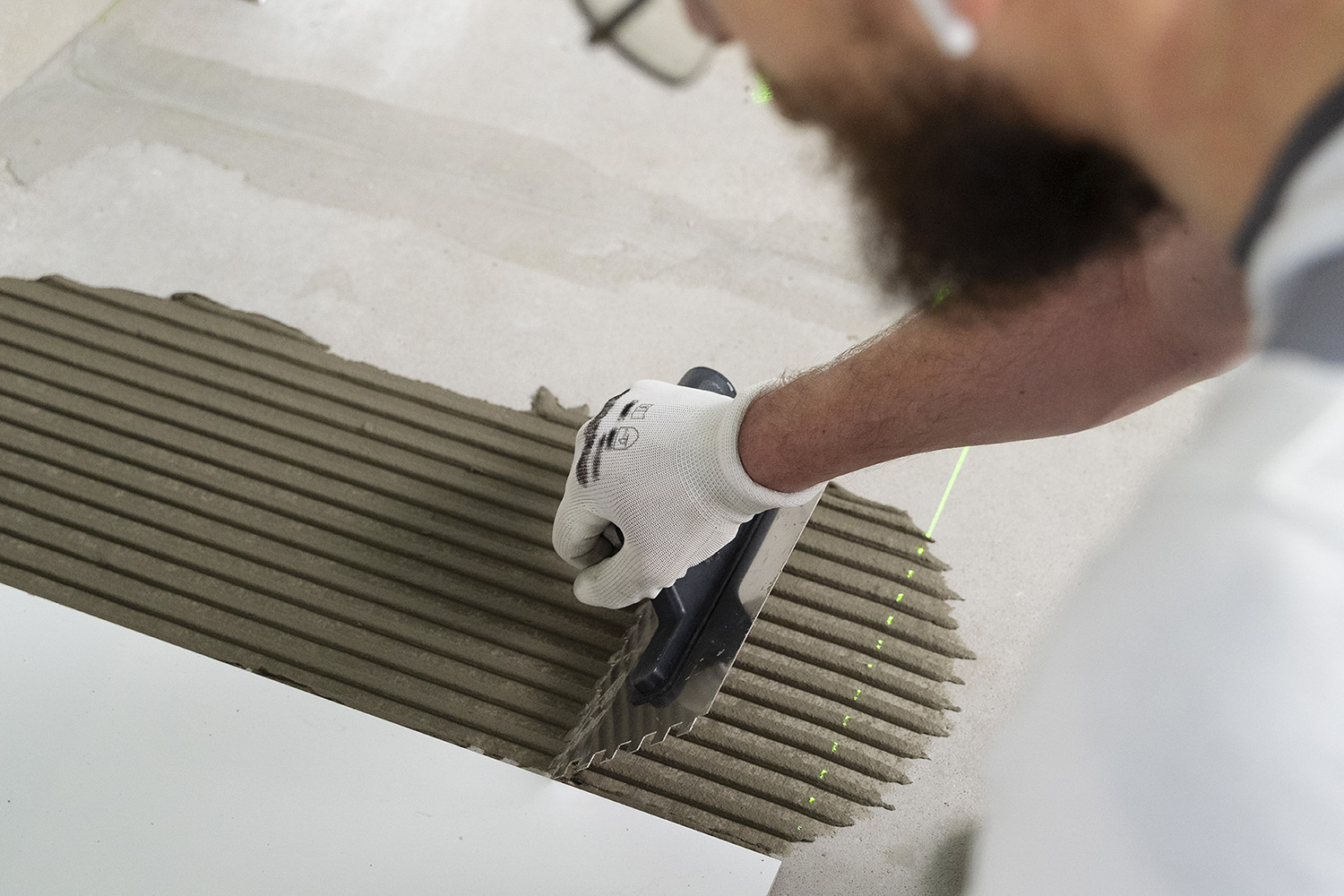In this landscape-format, professional-quality color photograph, a bearded Caucasian man is seen meticulously spreading a dark gray or brown cement-like compound over a white, flat surface, possibly plasterboard or floor tiles. This action creates a vertical line pattern, indicative of tile preparation or plaster application. The man, who has a long, curly, messy beard, is partially facing away from the camera, with the image taken over his shoulder. He is wearing black glasses, white earbuds, and a white shirt. His focus is on the task at hand, as evidenced by his right arm in the foreground, clad in a white glove, holding the spreading tool, and displaying the motion of the application process. The foreground is a bit blurry, drawing more attention to his detailed actions and the texture of the material being applied.